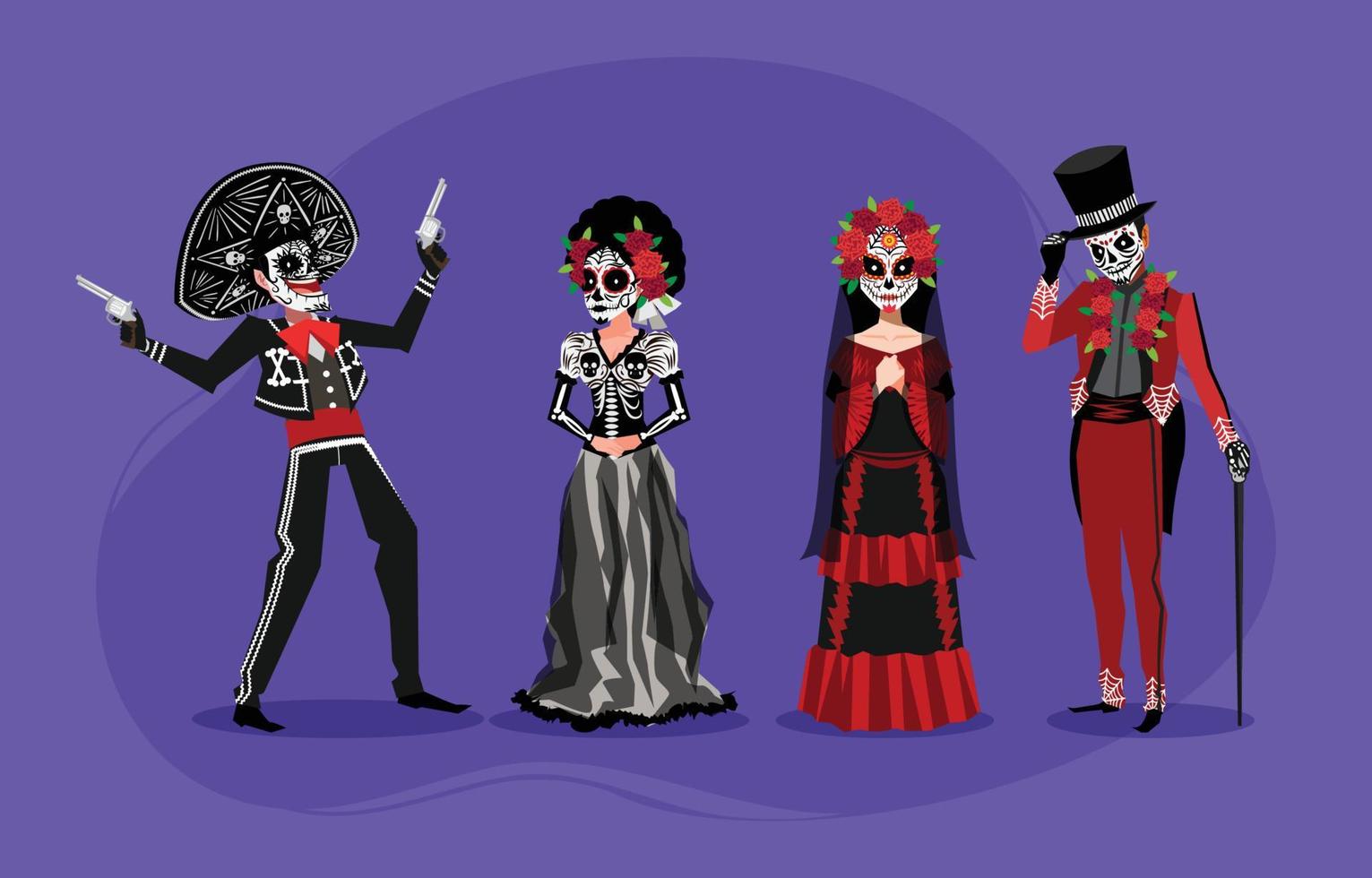Four cartoon characters are depicted in a vibrant artwork with a light and dark purple backdrop, celebrating Mexico's Day of the Dead. On the far left stands a joyous mariachi bandolero with a large black sombrero and a face painted like a skull. He brandishes two pistols in the air, adorned with gray metal and brown handles. Wearing black pants, a black jacket, and a red shirt, his outfit is completed with black shoes and a red tie. His face is further detailed with spider webs, suns, and black circles around his eyes.

Next to him, a woman with elaborate black hair, adorned with red and pink flowers and leaves, sports similar skull makeup. She is dressed in a black top featuring white accents and two skulls resembling a rib cage and spine. Her attire is complemented by a floor-length black and gray skirt with gray frills underneath.

The third character, another woman, also has her face painted in the same Day of the Dead style. She wears a striking red and black dress, a black veil, and flowers in her hair. Her black hair cascades down her sides, partially veiled.

Finally, the man on the right stands tall in a flamboyant red suit with coattails, a gray undervest, and a red top vest. His red pants feature white web patterns at the base, and he holds a black cane in his right hand, which is sheathed in a skeleton glove, matching the one on his left hand. A black top hat with a striped band completes his look, along with white webs on his red shirt and floral decorations around his neck. His facial paint mirrors the others, featuring intricate designs with red dots above his eyes.